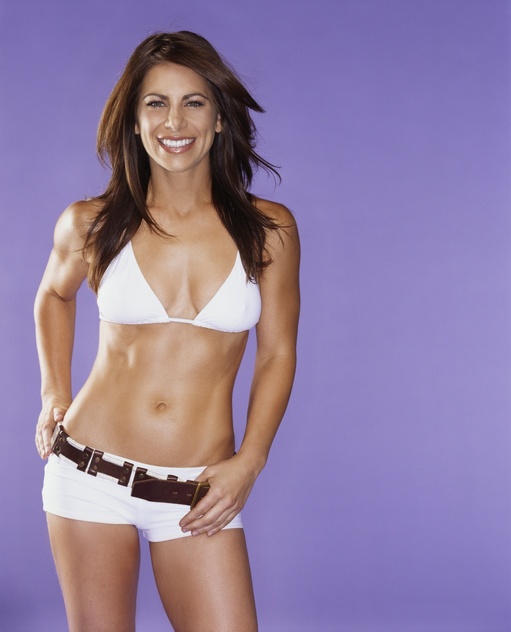The image depicts a strikingly fit woman, likely in her late 30s or early 40s, standing against a gradient purple backdrop that transitions from dark to light. She has long, black and brown hair that is feathered and styled to drape over her swimsuit straps. Her attire consists of a white bikini top paired with very short white shorts that feature a wide brown leather belt. She stands on the left side of the image, with her pose conveying confidence and poise; her right hand rests on her hip while her left hand, thumb hooked under the belt, is positioned in front of her. The photograph is cropped just above her knees, and the woman is smiling directly at the camera.